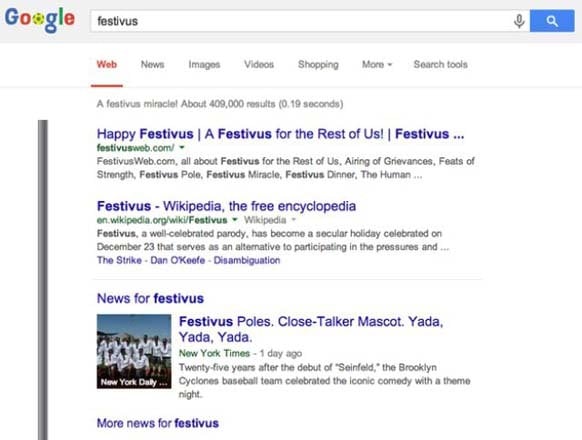This image captures a screenshot of a Google search bar displaying search results for "Festivus." The search yields the following key options: "Happy Festivus," "A Festivus for the rest of us," "Festivus - Wikipedia, the free encyclopedia," and a brief description of Festivus as a parody holiday celebrated on December 23rd as a secular alternative to Christmas, highlighting the pressures of traditional holidays. As a devoted Seinfeld fan who grew up watching the show, I am particularly familiar with Festivus. Originating from the sitcom, the holiday was created by Frank Costanza, George Costanza's father, as a replacement for Christmas, characterized by unique traditions like the "Airing of Grievances," where family members berate each other. Frank Costanza's irritable personality adds a humorous twist to this non-conventional celebration. The screenshot itself is square-shaped, perfectly framing the Google search interface.